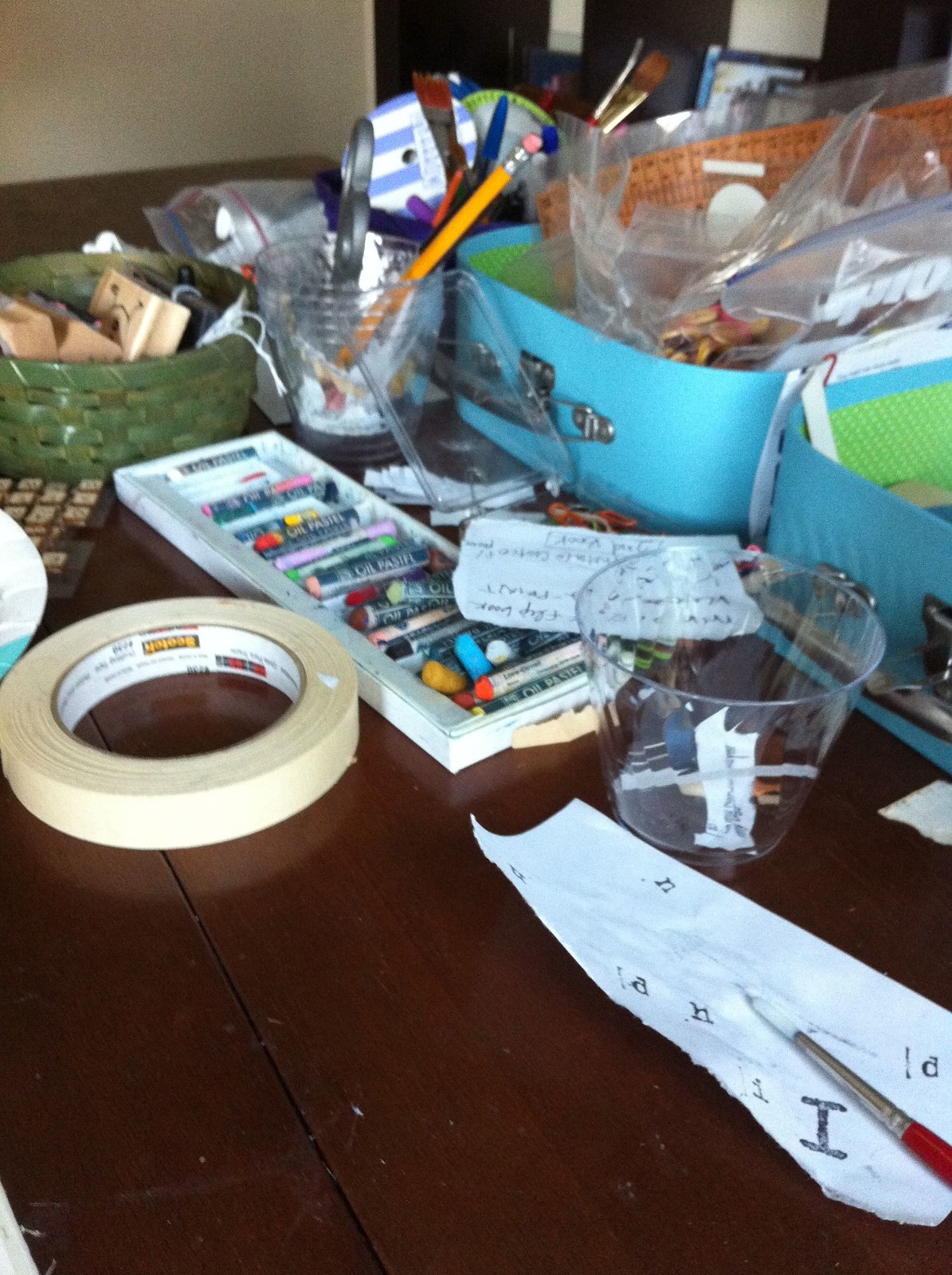The photograph depicts a cluttered arts and crafts table, which appears to be situated in a domestic setting, possibly a kitchen or study. The dark wooden table serves as the base for an assortment of office and craft supplies scattered across its surface. Prominently featured are clear plastic cups that hold a mix of items including a pencil and a pair of scissors. A roll of scotch tape can be seen alongside a bin filled with an array of colorful crayons. To the right side of the table, several blue rectangular metal bins contain larger, indistinguishable items.

On the left-hand side of the table, there's a woven green basket housing wooden blocks, one of which displays a face that could be either a smiley or a frowny face. In the foreground lies a torn piece of paper dotted with random letters, giving the impression of haphazard use rather than organized writing. The image, taken vertically, adds to the sense of a spontaneous snapshot, likely captured with a phone in portrait mode. The overall scene is characterized by a busy, creative atmosphere reflective of an active arts and crafts session.